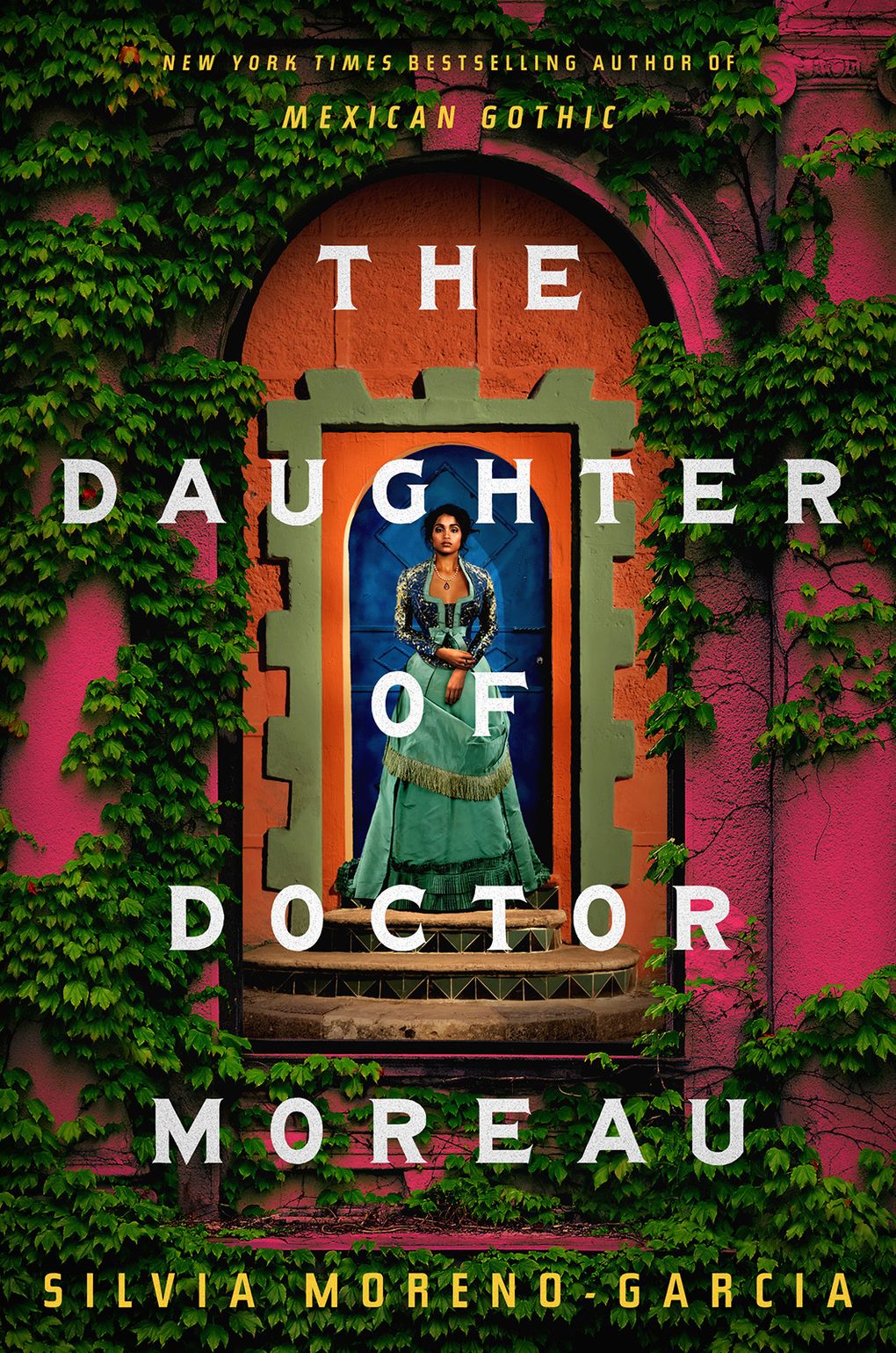The book cover features a colorful and intricate design, prominently showcasing a Hispanic or Latina woman standing in a doorway. The doorway is vivid blue and edged with a green geometric pattern, resembling a peephole shape. She is dressed in a detailed ensemble, featuring an elaborate green gown with fringe, a navy blue bodice accented with gold embroidery, and dark hair. The building in the background is a striking reddish-pink color with an orange door, entirely enveloped in green ivy. The title "The Daughter of Dr. Moreau" spans the middle of the cover in large white capital letters. At the top, in yellow font, it reads "New York Times bestselling author of Mexican Gothic," and at the bottom, also in yellow, is the author’s name, Silvia Moreno-Garcia. The overall composition exudes a sense of mystery and rich visual appeal.